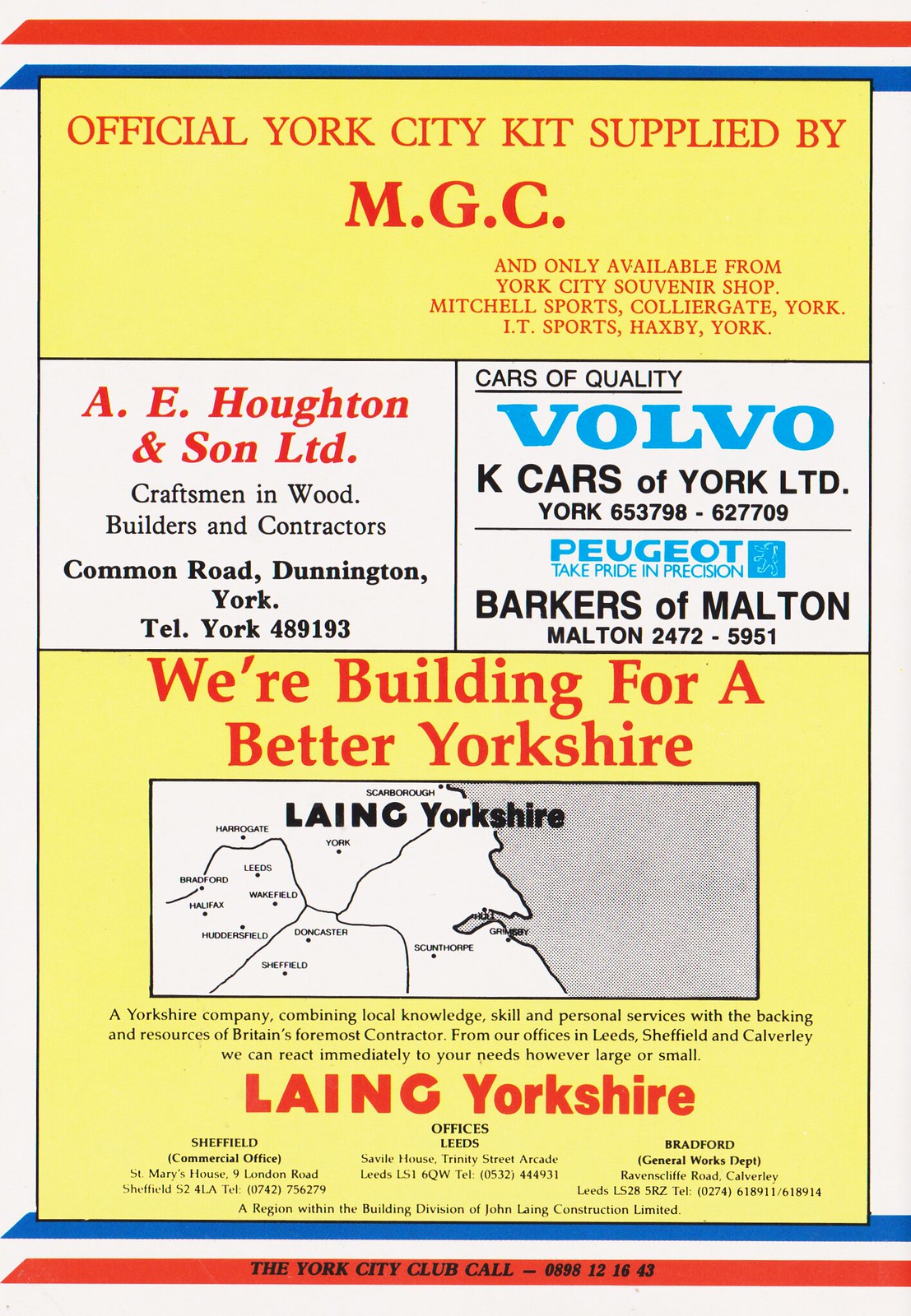This image depicts a tall, rectangular vintage advertisement poster set against a white background. The design prominently features red and blue stripes across the top and bottom edges. In the center of the poster, there is a prominent yellow rectangle with red text at the top that reads: "Official York City Kit Supplied by MGC, and only available from York City Souvenir Shop, Mitchell Sports, Colliergate, York, IT Sports, Haxby, York."

Below this text, the poster displays two white advertisements side by side. The left ad is for "A.E. Hooten & Son Ltd, Craftsmen in Wood, Builders and Contractors, Common Road, Dunnington, York, Telephone, York 489193," written in red. The right ad is for "Cars of Quality, Volvo" and also mentions "Pugot, Take Pride in Precision, Barkers of Malton, Malton 2472-5951," written in blue.

At the bottom of the yellow rectangle, it reads in red text, "We're Building for a Better Yorkshire." Below this, there is a black and white map of Yorkshire followed by additional black text providing locations for offices.

Overall, this poster combines vibrant colors and structured advertisements to present an engaging promotional design that highlights local businesses and their offerings.